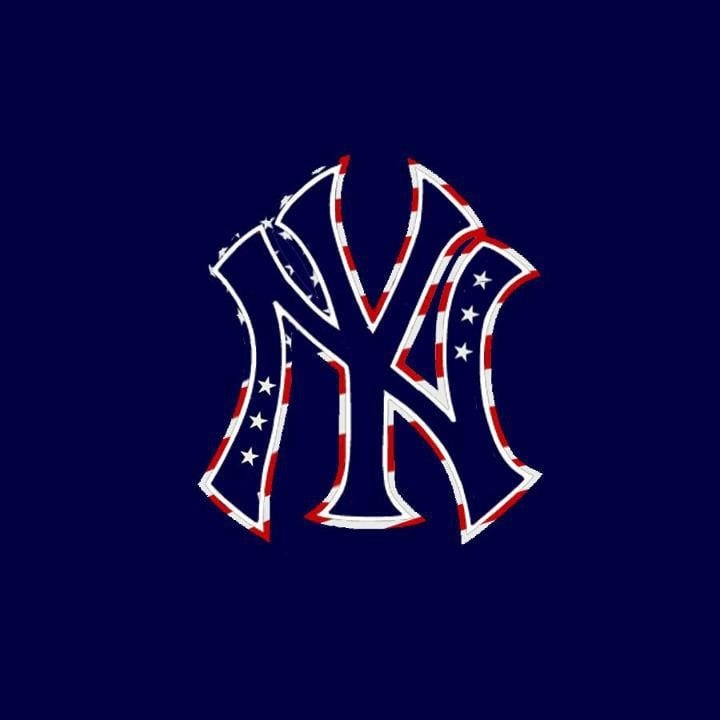The image features a stylized New York Yankees logo set against a dark navy blue background. Central to the composition is a capital "NY," where the "N" is positioned slightly in front of the "Y." Both letters exhibit significant curvature, with the "N" appearing rounded and twisted and the "Y" displaying similar curvature at its ends. The "NY" is outlined in white and filled with an American flag design. The left side of the "N" contains three white stars, mirrored by three more on the right side, symbolizing the stars on the flag. Red and white stripes run through both letters, emulating the American flag’s stripes. The background and the colors used in the "NY" logo—navy blue, white, and red—reinforce the American flag theme. There are no additional elements or text in the image, making the stylized "NY" logo the focal point against the simple dark blue backdrop.